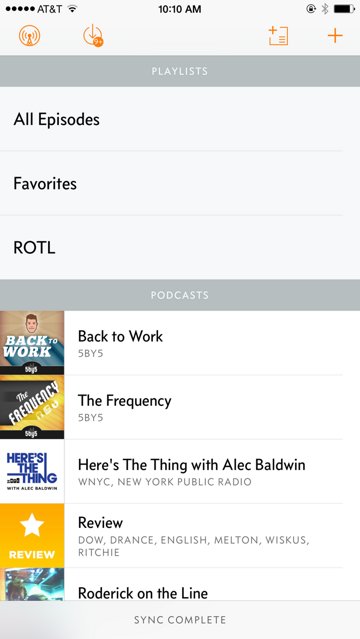This is a detailed screenshot taken from an iPhone, evidenced by several indicators typical of the iOS interface. At the top center of the screen, the time is displayed as 10:10 AM, reflecting a 12-hour format. In the top left corner, the carrier is shown to be AT&T with full signal strength bars. Adjacent to this, the Wi-Fi icon indicates a signal strength of about half. The top right corner of the screen features additional icons: a lock symbol indicating screen orientation lock, a grayed-out Bluetooth icon showing that Bluetooth is on but not connected to any devices, and a battery icon suggesting an approximate charge level of 80%.

Below these status indicators, there are several selectable options. The screen prominently displays options labeled as "Playlists," "Podcasts," and a status message stating "Sync Complete."

Under the "Playlists" section, three additional options are listed: "All Episodes," "Favorites," and an abbreviation, "ROTL."

Directly beneath these, within the "Podcasts" section, several podcast titles are visible:
- "Back to Work by 5by5"
- "The Frequency by 5by5"
- "Here's the Thing with Alec Baldwin by WNYC and New York Public Radio"
- "Review by Dow, Drance, English, Melton, Whiskas, and Ritchie"
- "Roderick on the Line"

This thorough capture encapsulates both the current system status and content options available to the user on their iPhone.